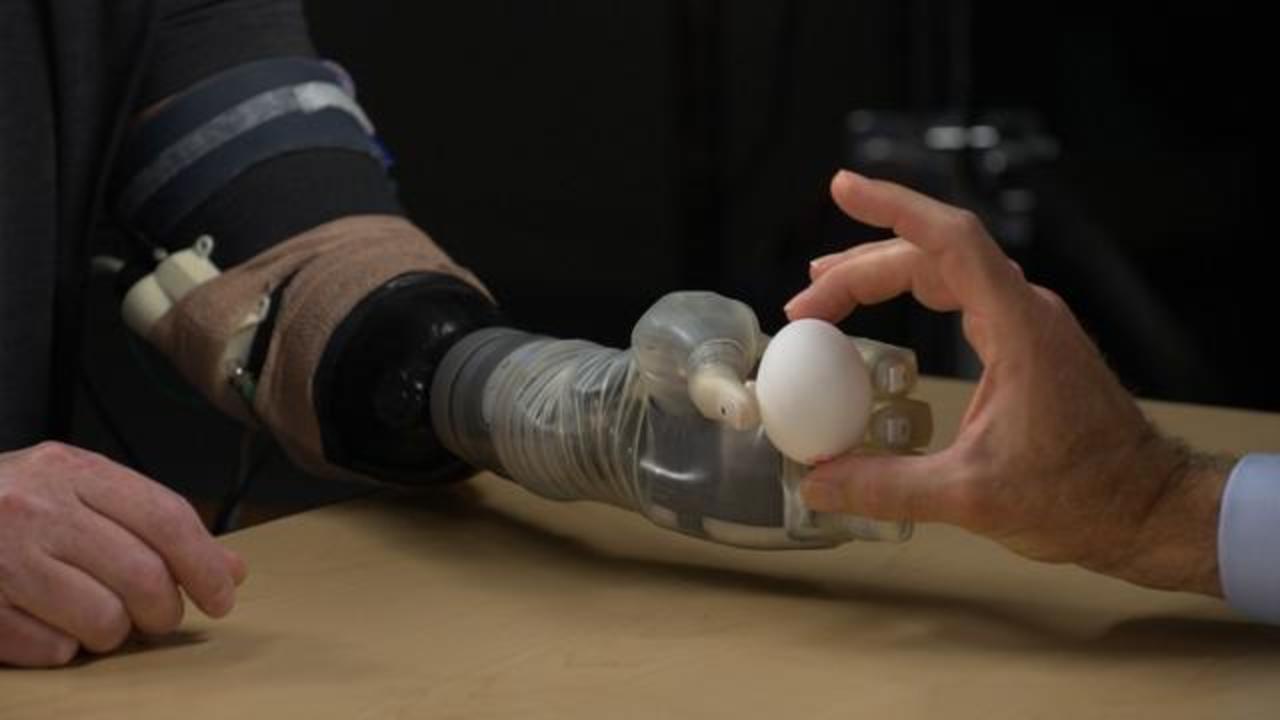A detailed description of the image shows a person sitting at a light-colored table, equipped with a prosthetic, highly-advanced robotic arm extending from the elbow to the hand. This prosthesis features a combination of silicone, hard plastic, and metallic elements, with intricately designed fingers and visible wiring. The hand, which has a partially gray and black coloration, is reaching to grasp a white chicken egg being handed to them by another individual across the table. The second individual, who is wearing a lab coat, is assisting in what appears to be a test of the prosthetic's functionality. The background is draped in a black curtain or cloth, providing a stark contrast that highlights the interaction and the high-tech nature of the prosthetic device.